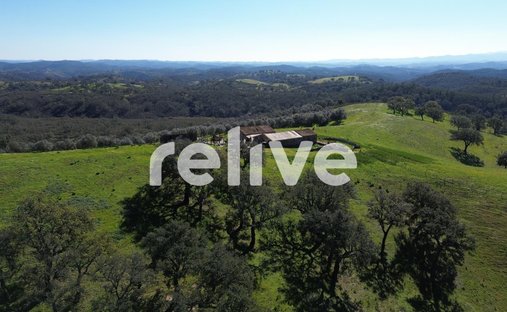The image captures a serene outdoor scene bathed in daylight, featuring lush green hills dotted with occasional trees and an expansive grassy landscape. The sky overhead is a clear, vibrant blue, emphasizing the freshness of the day. Central to the landscape is a quaint structure with a brown roof accompanied by sections of white, harmoniously blending with the natural surroundings. Superimposed in the middle of the image, in a stylish lowercase font, is the word "Relive" spelled R-I-L-I-V-E, subtly yet distinctly standing out. This captivating blend of text and landscape evokes a sense of tranquility and renewal.